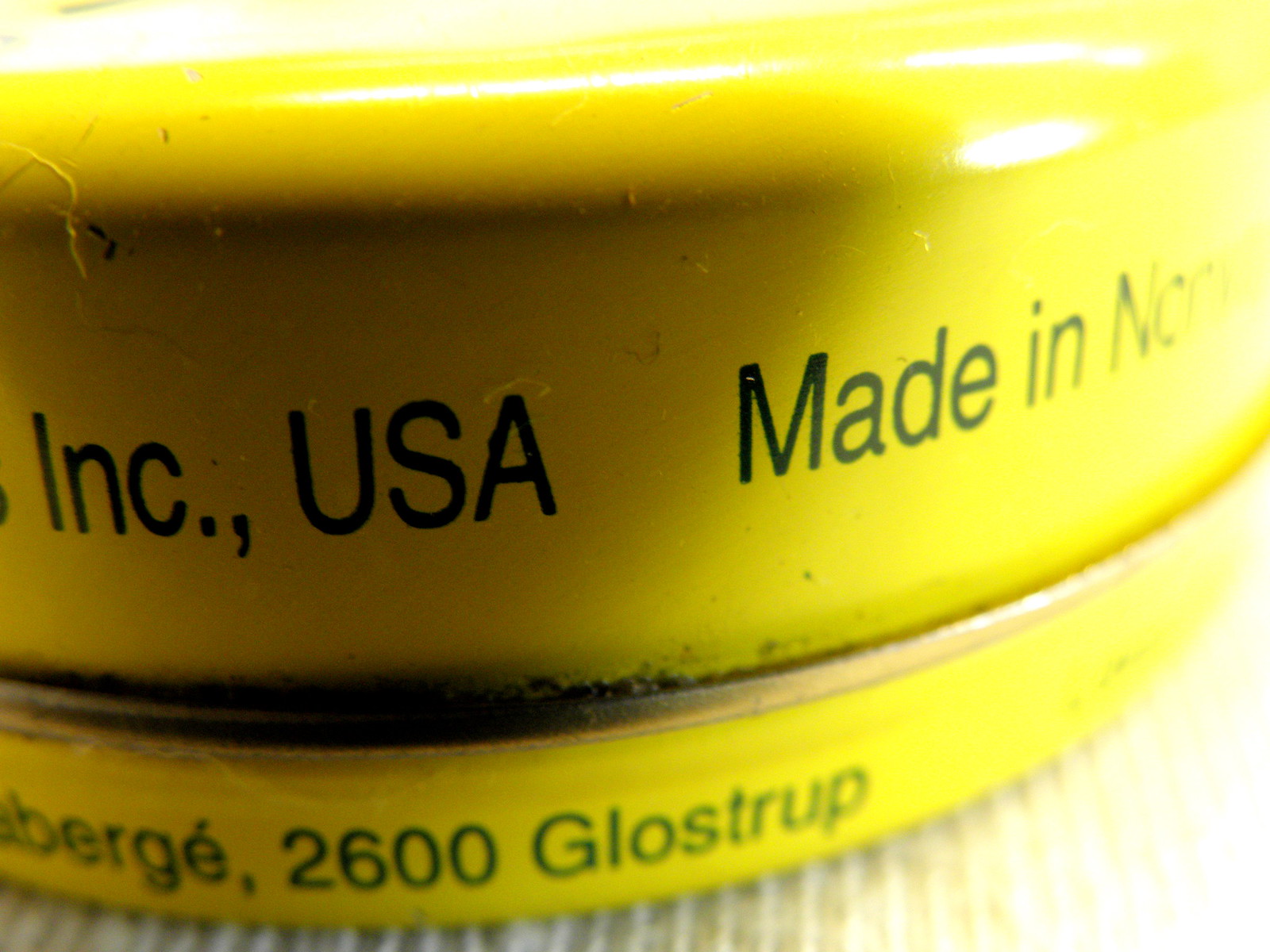The image depicts a close-up of an old, bright yellow metal tin, likely used for storing items like lip balm or cream. The tin is very shiny on the top but shows signs of wear and matte texture on the sides. It is set on a stark white background, which accentuates its vibrant color. The lighting comes from the top right, casting distinct shadows to the left and causing some overexposure on the right side, which washes out detail in that area.

The tin bears black text that reads "Ink, USA" near the top, and beneath that, partially visible, "made in" followed by "N-O-R," suggesting it might be from Norway. Further down, in green lettering, it shows "BER-." followed by a partial address "-2600 Gloucester" and what appears to be "Gloss strip" likely meant to be "Glostrup," indicating some connection to a place or manufacturer. The rim around the tin is silver, with various chips indicating its age and usage.